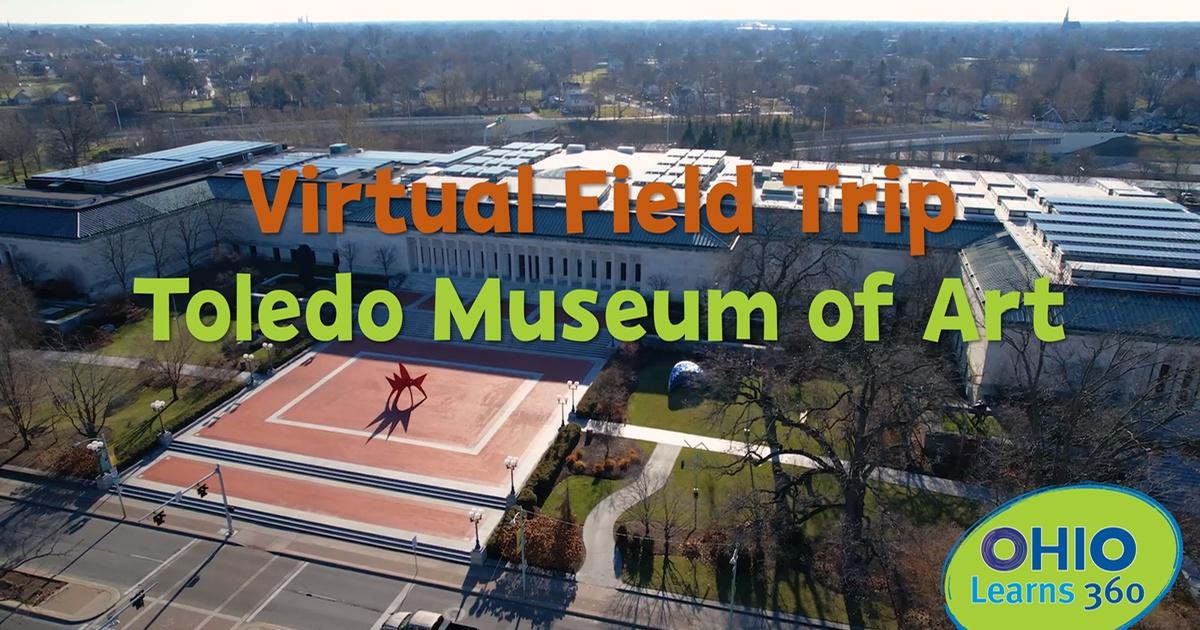The image depicts a virtual field trip offering for the Toledo Museum of Art. The centerpiece is the museum's edifice, a white building with a gray-topped roof. Above the image, bold text reads "An Armature Virtual Field Trip," indicating the tour nature of the content. Beneath it, a green banner displays "Toledo Museum of Art" in distinct text. In the bottom right corner, partially cut off, is a green oval edged in blue, featuring the text "Ohio Learns 360." The first 'O' in Ohio is purple, and the rest of the letters are blue. The background features a pale sky with a white hue, complemented by a line of trees with sparse foliage, suggesting it may be fall or winter.